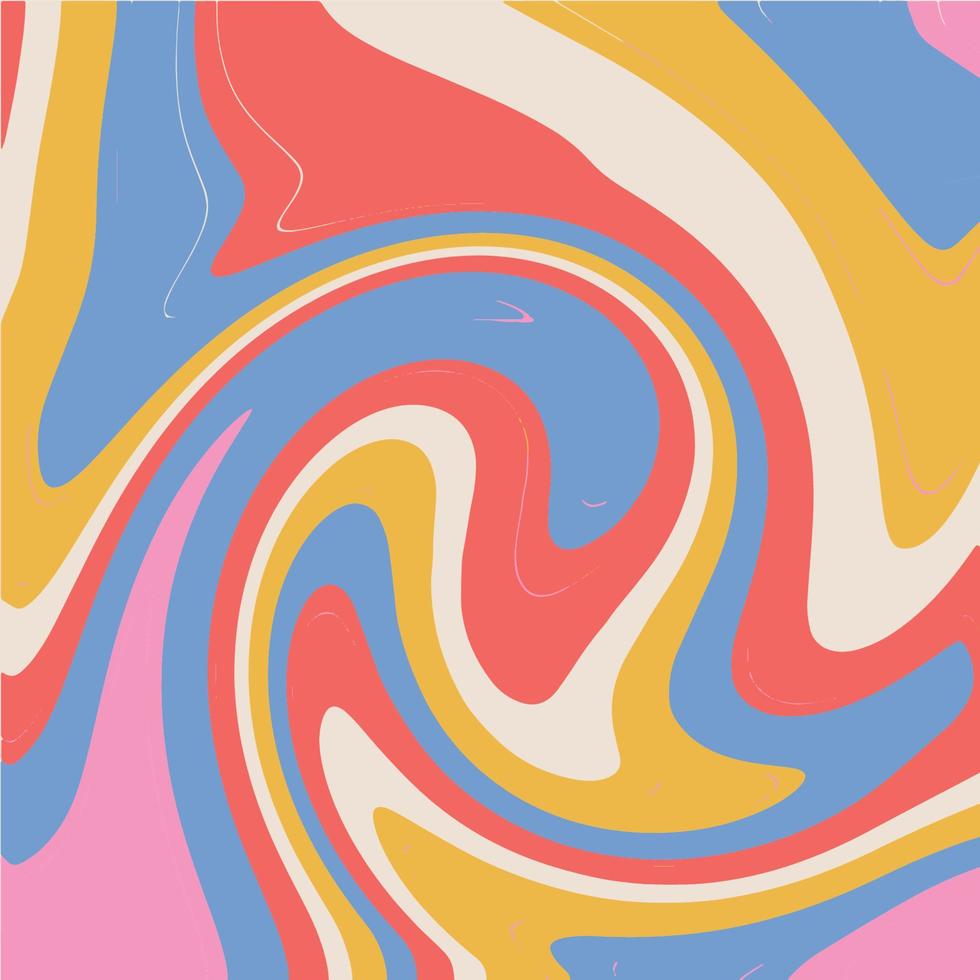This image is a vibrant, abstract illustration that embodies a psychedelic 1970s retro style. The square format artwork features a captivating swirl pattern, showcasing a rich palette of colors including a warm, dark yellow, eggshell white, light red, pink, light blue, cream, gold, and orange. The hues are distinctly separated, avoiding any blending, yet they swirl independently in a harmonious manner. The composition includes a strong diagonal stripe extending from the top center to the mid-right section. Additionally, a dynamic swirling shape rises from the bottom left corner and curves around the center, giving the piece an intricate and engaging flow. The overall appearance of the design maintains a flat, digital art feel, emphasizing its abstract nature.